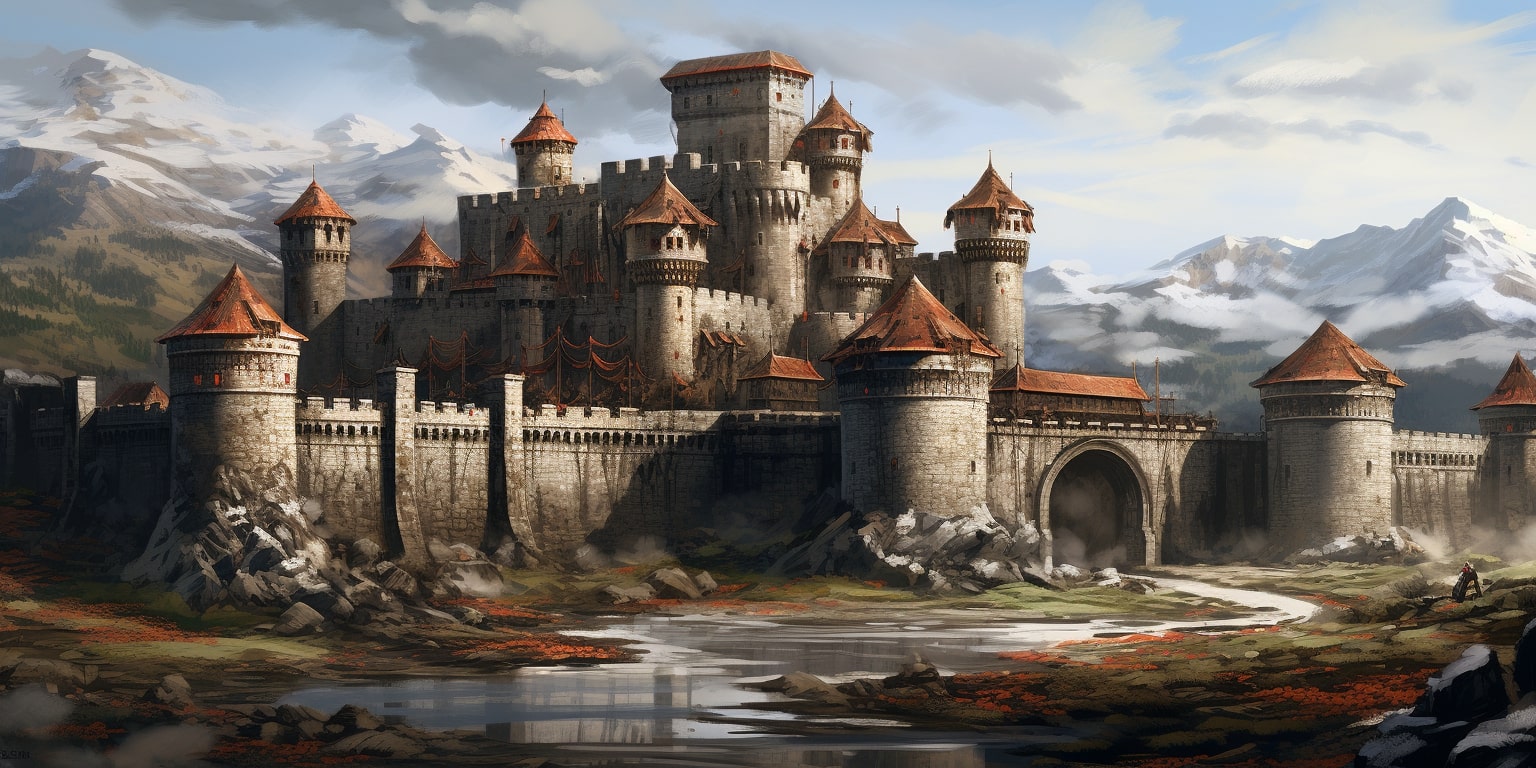This detailed painting depicts a large medieval castle set against a backdrop of softly painted mountains beneath a light blue sky dotted with clouds. The castle, constructed with predominantly gray stone, is characterized by numerous cylindrical towers topped with cone-shaped roofs in striking red or brownish-orange hues. The castle's formidable structure includes a surrounding protective wall punctuated by at least four visible watchtowers. A moat, perhaps somewhat dried up, runs along the front of the castle, its water glistening under the harsh lighting. The entrance to the castle appears to be a gaping hole, an ominous and grand gateway. To the right, one can spot a solitary figure seated, adding a touch of life to the otherwise sparse human presence. Additionally, the surrounding landscape features red foliage, contrasting vividly with the castle's somber tones, enhancing the scene's surreal atmosphere.